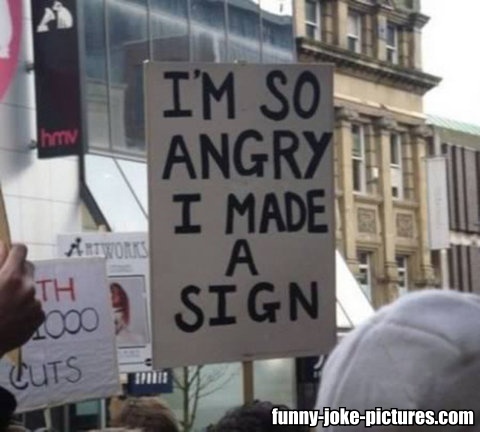This image captures a lively protest rally set against a backdrop of older, four to five-story apartment buildings and a cityscape that includes what appears to be an electronics store. The central focus of the image is a protest sign held prominently in the middle, with bold capital black letters that read, "I AM SO ANGRY, I MADE A SIGN." Surrounding this main sign are at least two other partially obscured signs; one of these has the word "cuts" visible at the bottom, and the other seems to include a picture of some kind. The heads of several protesters and a single hand holding a sign are visible in the foreground, emphasizing the crowd's density. On the bottom right corner of the image, the text "funny-joke-pictures.com" is clearly written in white letters, indicating the source of the photo.